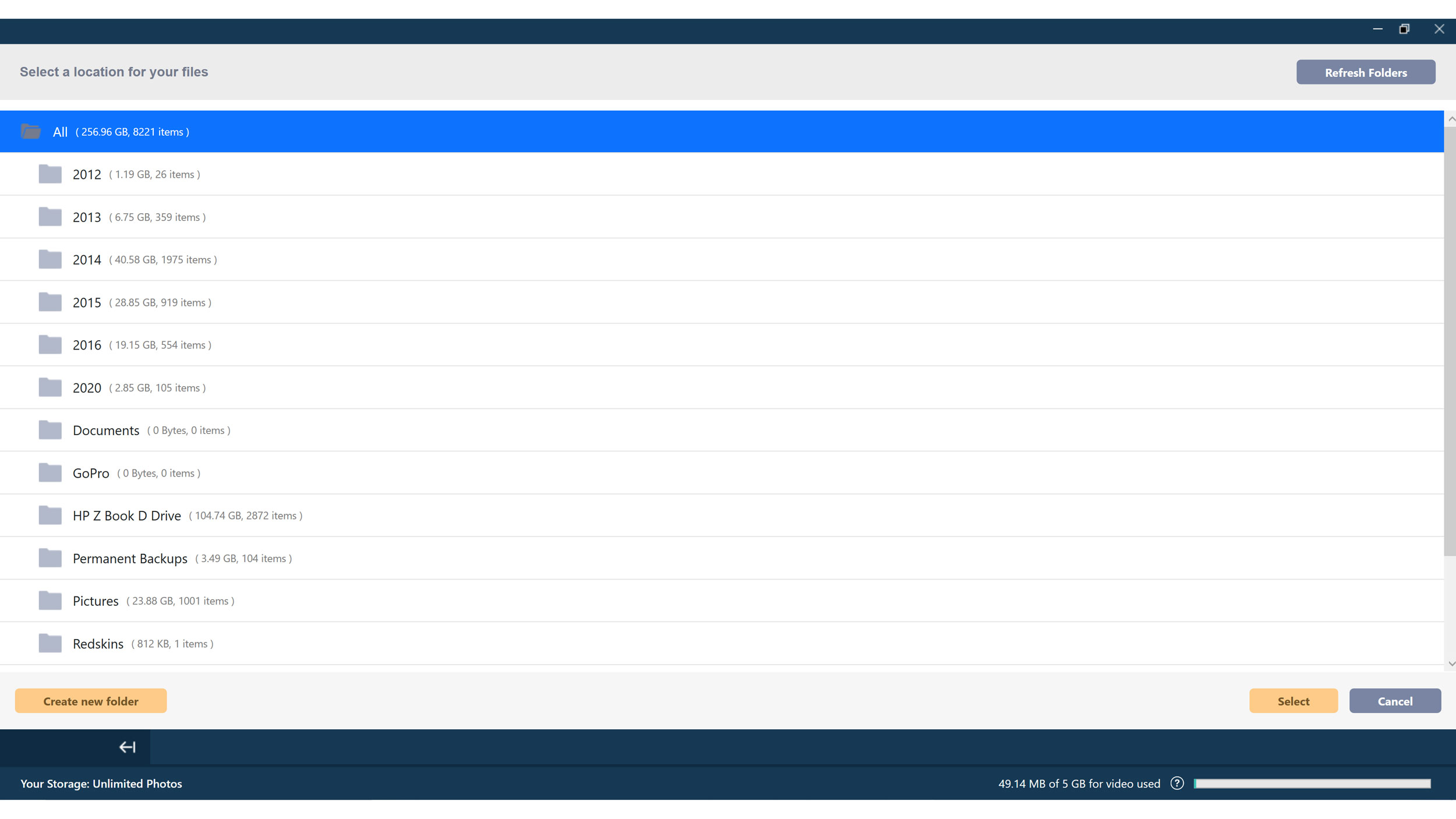Screenshot of the backend interface of a website or application displaying a structured list of folders. At the top, a dark blue title bar showcases three familiar Windows control buttons—Minimize, Maximize, and Close—located on the right side. Directly beneath the title bar, a gray navigation bar splits into two sections: "Select a location for your files" on the left and "Refresh Folders" on the right.

The main section below the navigation bar features a hierarchical list of folders, each accompanied by a folder icon. The list starts with "All" at the top, implying a comprehensive view, followed by folders labeled sequentially by year from 2012 to 2020. The structure continues with additional directories named "Documents," "GoPro," "HP," "ZBook," "D-Drive," "Permanent Backups," "Pictures," and "Redskins."

At the bottom of the screen, another gray bar spans the width, offering three action buttons. On the left side, a yellow "Create New Folder" button stands out. On the right side, blue "Select" and gray "Cancel" buttons are positioned next to each other, providing options to finalize or discard the current operation.